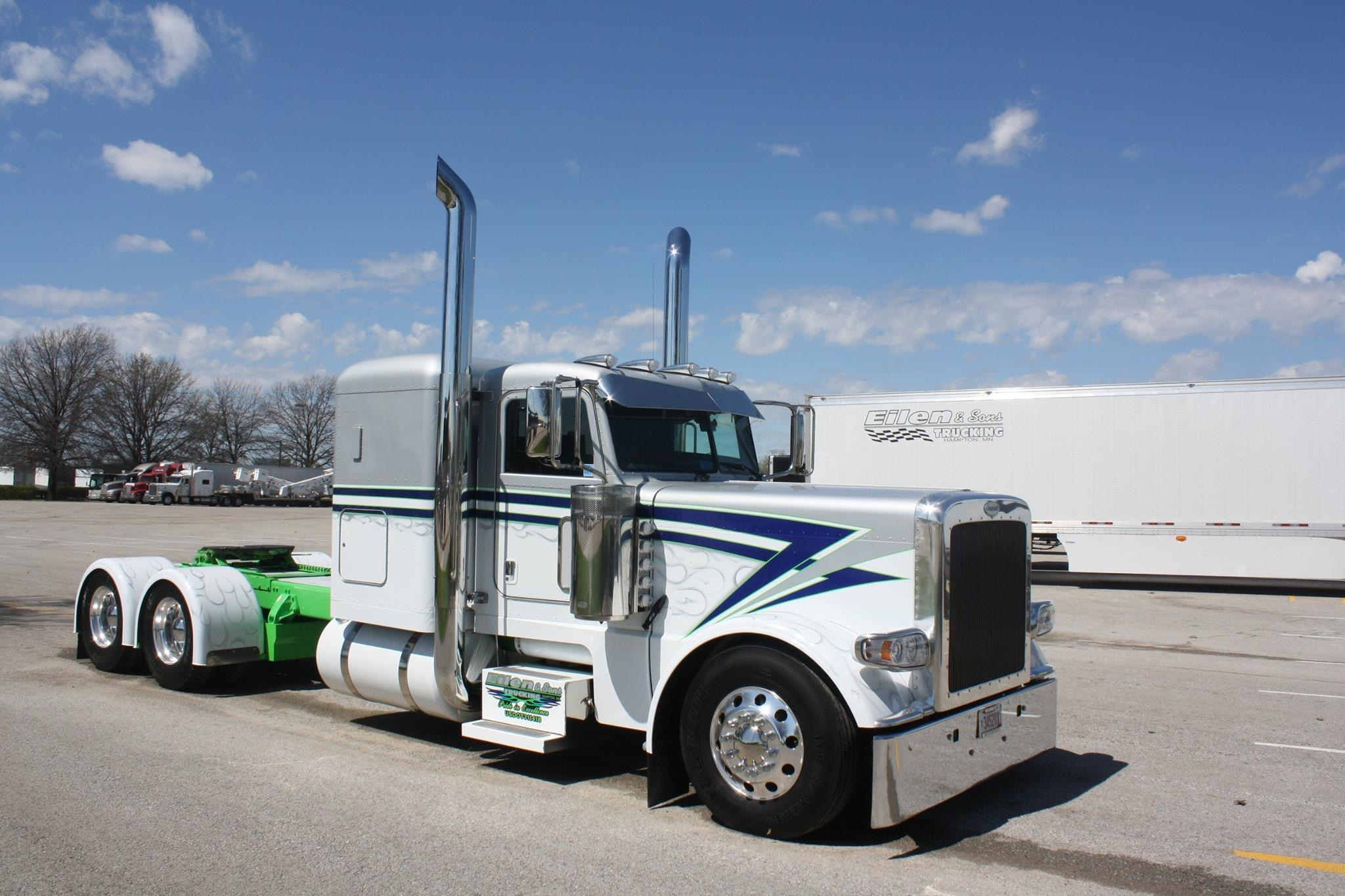This is a detailed color photo capturing a semi-truck parked in a lot without its trailer. The semi-cab, facing to the right, presents a two-tone appearance with a matte aluminum gray top half and a white bottom half. Notably, it features prominent blue stripes and a striking lightning bolt design across the middle, composed of two blue streaks with a green outline. The rear section of the truck, where the trailer attaches, is vivid neon green and partially covered by white wheel covers. The vehicle is equipped with two tall, highly reflective chrome smokestacks, adding a polished look to its robust structure. The background includes another semi-truck with a trailer displaying "Island and Sons Trucking," as well as several other semi-tractors, some potentially connected to their trailers. The truck also includes visible steps and hint of sleeping quarters.